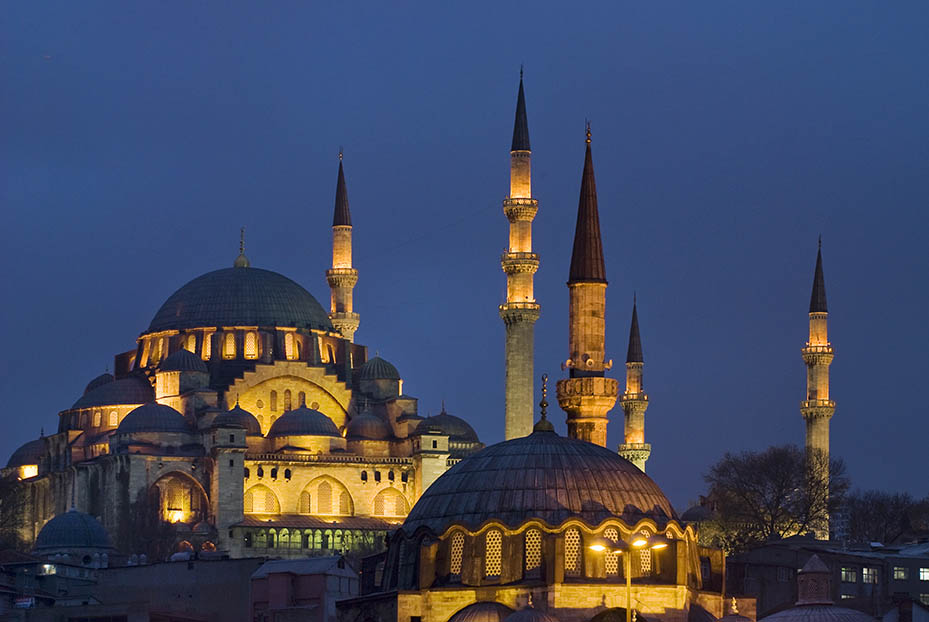This photograph captures a stunning scene of Middle Eastern architecture at twilight, possibly depicting a mosque. The image is dominated by two ornate buildings with domed roofs, reminiscent of the style of the Taj Mahal. The domes exhibit scalloped edges and are surrounded by rows of brightly lit windows, casting a golden glow. Both buildings feature archways and intricate brickwork, making them appear highly ornamental. In the background, five slender, spiked towers elevate into the deepening blue sky, each tipped with pointed cones, while lights adorn the towers and buildings, creating a spectacular nightscape. Foreground details include low buildings in shadow, deciduous trees, and glass doors on the main structure. The scene is bathed in twilight's darker blue hues, adding to the overall ambiance. The ornate architecture, with its domes, arches, and illuminated windows, stands out vividly against this backdrop.